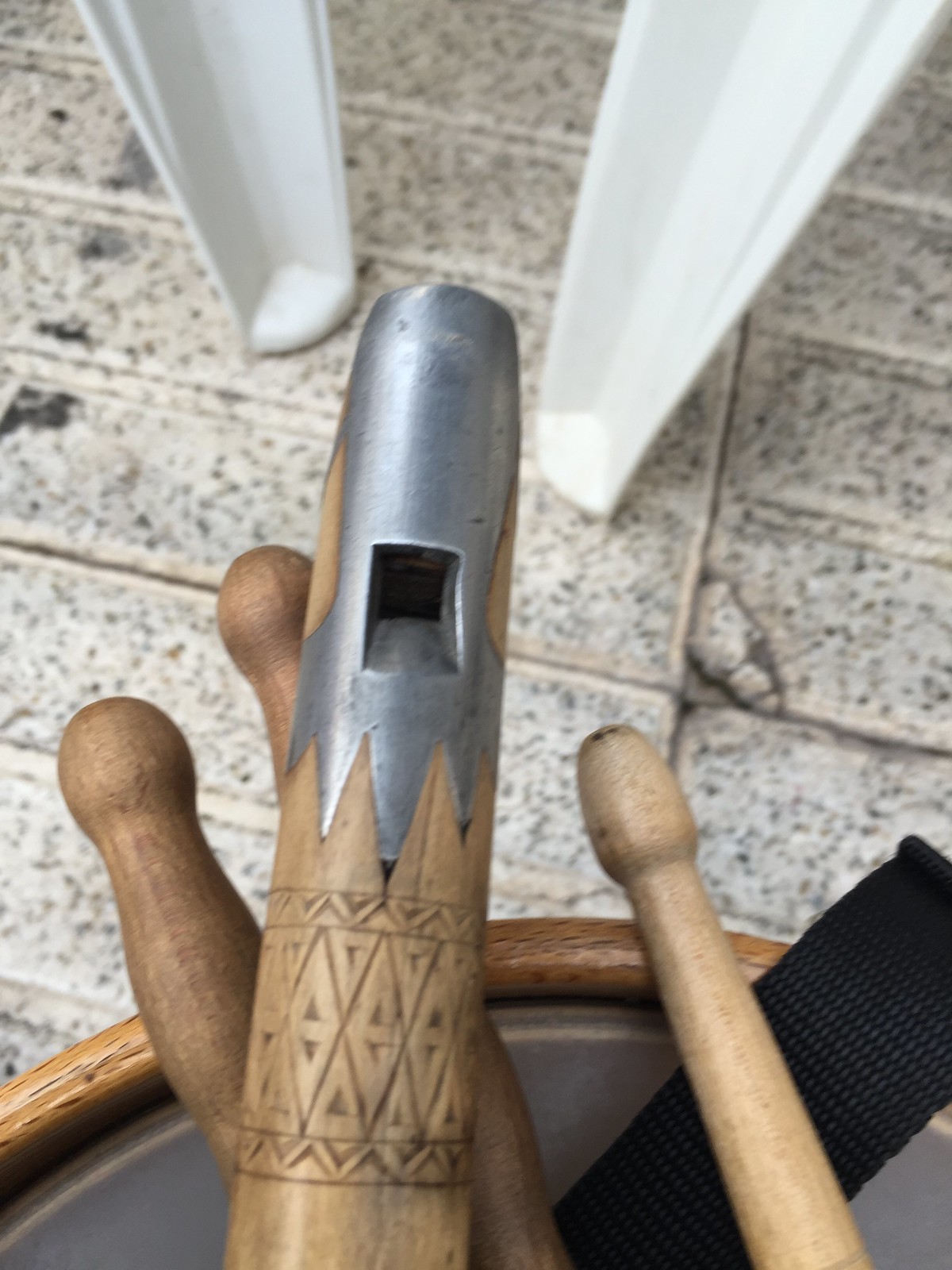The image is a detailed, up-close photograph of a wooden musical instrument, possibly a reed or flute, with intricate diamond-shaped carvings and a distinctive silver tip featuring an air hole and silver triangular embellishments. The instrument is lying on three wooden sticks that resemble drumsticks. In the lower right corner, there is a black cloth strap partially visible beneath one of the sticks. The background features a tan, black-speckled tiled floor, which appears slightly cracked, and the partially visible legs of a white plastic table or chair.